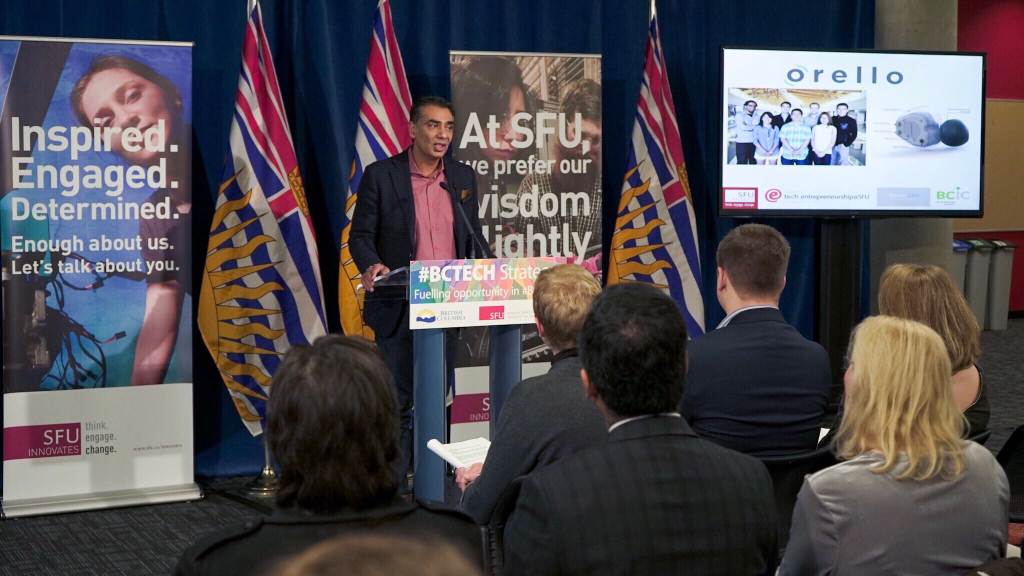In an image captured from the back of a room, we see a formal meeting in progress with an audience composed of people in suits attentively facing a podium. The speaker, a man with short dark hair in a dark suit coat and pink shirt, stands behind a blue podium adorned with a sign that reads "#BCTechStrategy: Fueling Opportunities." Behind him, three flags depict a red, white, and blue design with yellow suns. To his left is a banner inscribed with, "Inspired, Engaged, Determined. Enough About Us, Let's Talk About You," under the SFU logo. Another sign to the right says, "At SFU, we prefer our wisdom..." partially obscured. Additionally, a TV screen to the right displays the word "Orello" with an image of people standing facing the camera. The room is filled with a mix of men and women, emphasizing a professional setting possibly related to a college or a tech strategy event.